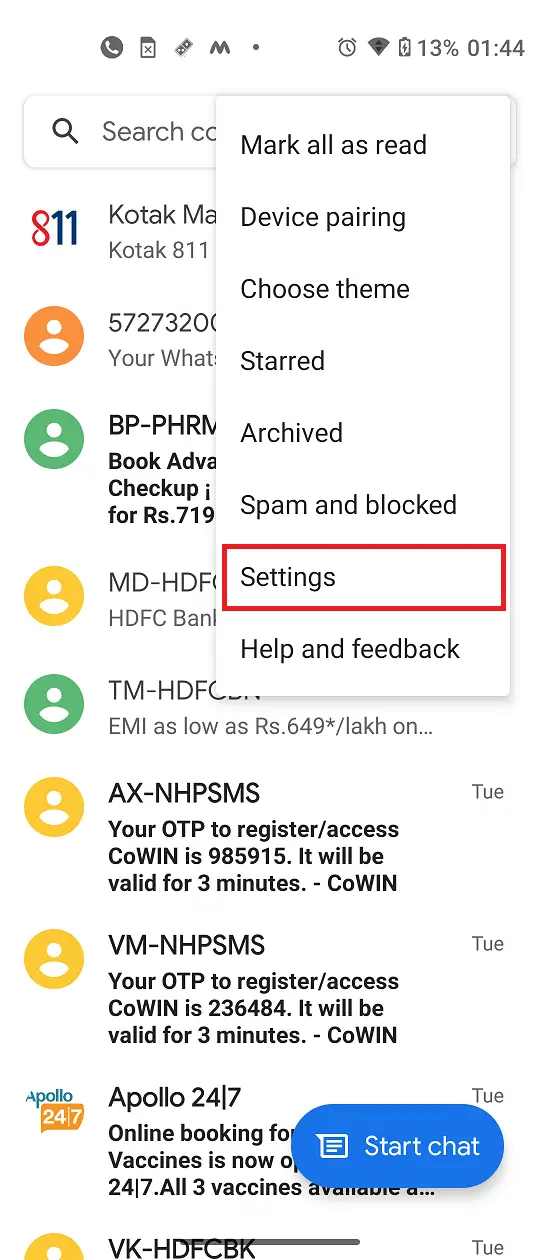In the upper left-hand corner of the image, there's a small circle that might contain a phone icon, though it's hard to discern due to its size. Adjacent to this circle is a box displaying a letter. Further to the right, there are various icons and text elements: the letter "M" followed by a dot, a clock, a Wi-Fi symbol, and a battery indicator showing 13%. Nearby, the time is displayed as "01:44".

Below these elements, much of the content is obscured by a prominent white rectangle. Visible text within this area includes options such as "Mark all as read," "Device pairing," "Choose theme," "Starred," "Archived," "Spam and blocked," and "Settings," with "Settings" outlined in a red rectangle. Additionally, "Help and feedback" is visible.

To the left of the image, more details emerge from beneath the white rectangle: the date "8-11" is displayed along with several colored circles, each with a person icon inside. The circles are in orange, blue, yellow, green, and more yellow. Next to these, it says "Apollo 24-7." Although many details are blocked by the white rectangle, some of the hidden text can be inferred.

Finally, at the bottom right, there's a blue button featuring a speech bubble with horizontal lines inside, accompanied by the words "Start Chat."